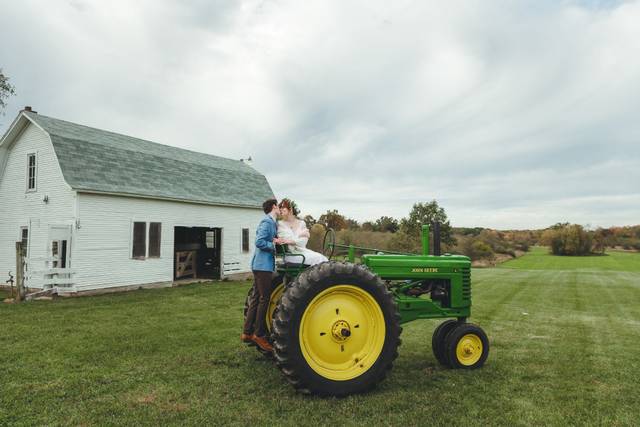In this idyllic outdoor post-wedding photograph, a newlywed couple captures a tender moment on a green John Deere tractor set in a verdant farm field. The scene is dominated by the iconic green and yellow of the tractor, with its large back wheels and smaller front wheels. The bride, resplendent in a white wedding gown and adorned with a floral wreath in her hair, sits gracefully on the tractor seat. She is turned sideways, looking back to share a kiss with the groom, who stands on the tractor step. He is smartly dressed in a blue suit jacket, dark brown pants, and light brown dress shoes. In the background, a picturesque white barn with a gabled roof painted in shades of gray adds rustic charm to the composition. One of the barn doors is open, revealing a glimpse of wooden pallets inside. The scene is further framed by a cloudy gray sky with wisps of light blue and fluffy clouds, and framed by distant trees and brush, emphasizing the couple’s intimate, solitary moment amidst nature.